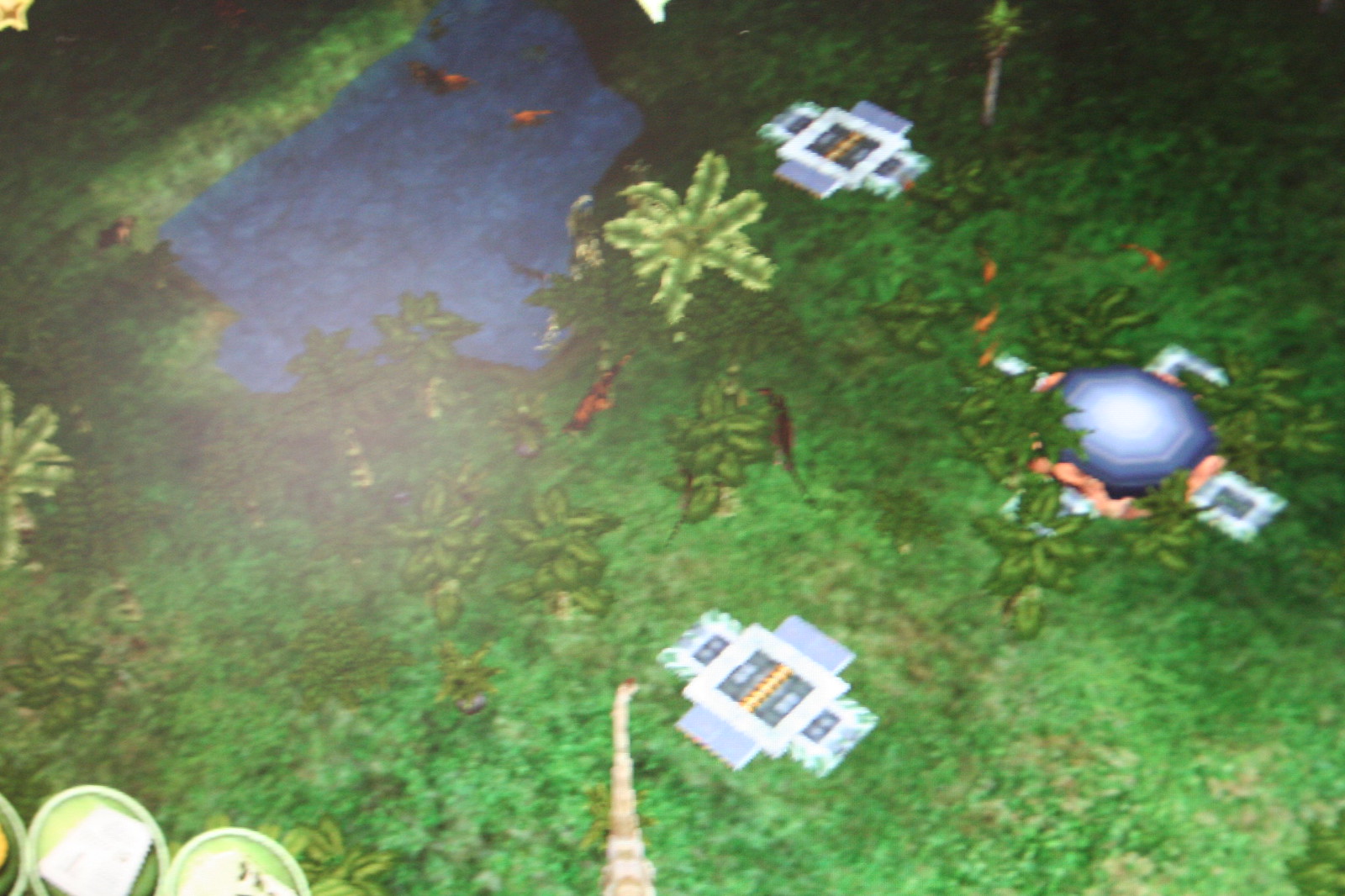This is a large, square screenshot from a video game that appears dark and grainy, with colors not looking very vivid. The image is an overhead view of a jungle-like environment. There are three distinct structures: one located at the bottom center, and two on the left side of the image.

The overall environment features dense grass and trees, suggesting a wild, untamed setting. In the image, a long, narrow neck resembling that of a dinosaur stretches towards the left, evoking imagery typical of a Jurassic Park-themed game. Further reinforcing this theme, the center of the image showcases smaller versions of what look like T-rexes.

On the left side, slightly towards the center, stands a round, dome-shaped building. Near the bottom center of the image is a square structure. Additionally, at the top left, there's a small pond with animals swimming in it, contributing to the lively and wild atmosphere of the scene.